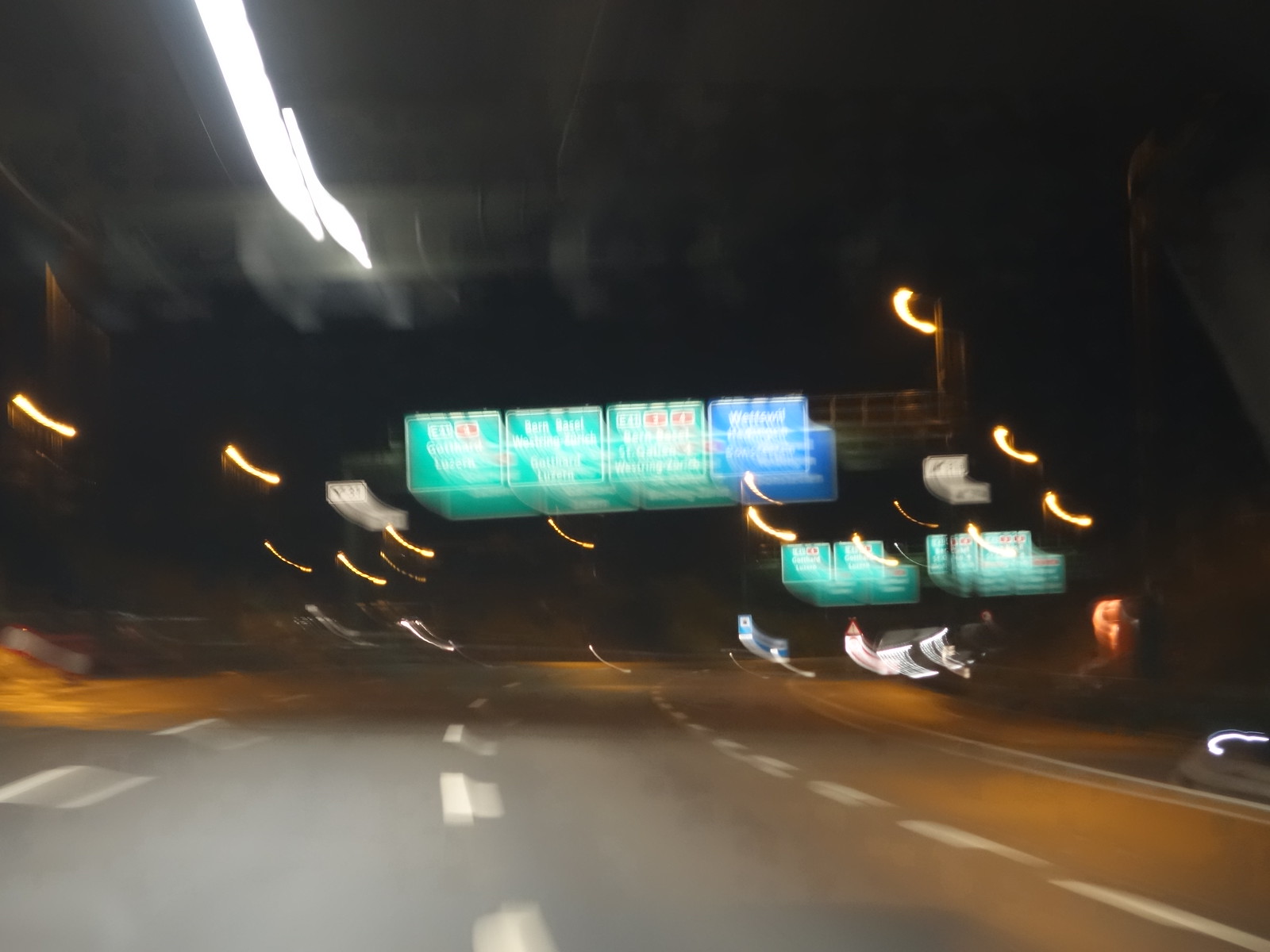The photograph captures an extremely blurry and motion-distorted scene of a highway at night, likely taken from a moving car. The sky looms as an inky black void, dotted with a curvy motion blur of street lamps that create squiggly lines due to the car's movement. The highway itself appears to be large, possibly a freeway with at least four lanes divided by white broken lines that, despite the blur, are relatively more distinct. Overhead, green highway signs dominate the scene, hanging from beams with text that is unreadable due to the blur; a single blue sign is also present among them. The road showcases a gray paved texture, and its white stripes display a motion blur effect, yet they remain clearer than the signs and lights. A bright light descends from the top left of the image, further contributing to the double vision and stigmatism-like effect observed in the photograph. The image is pervaded by reflections, possibly from a windshield, adding another layer of distortion to this chaotic nighttime highway scene.